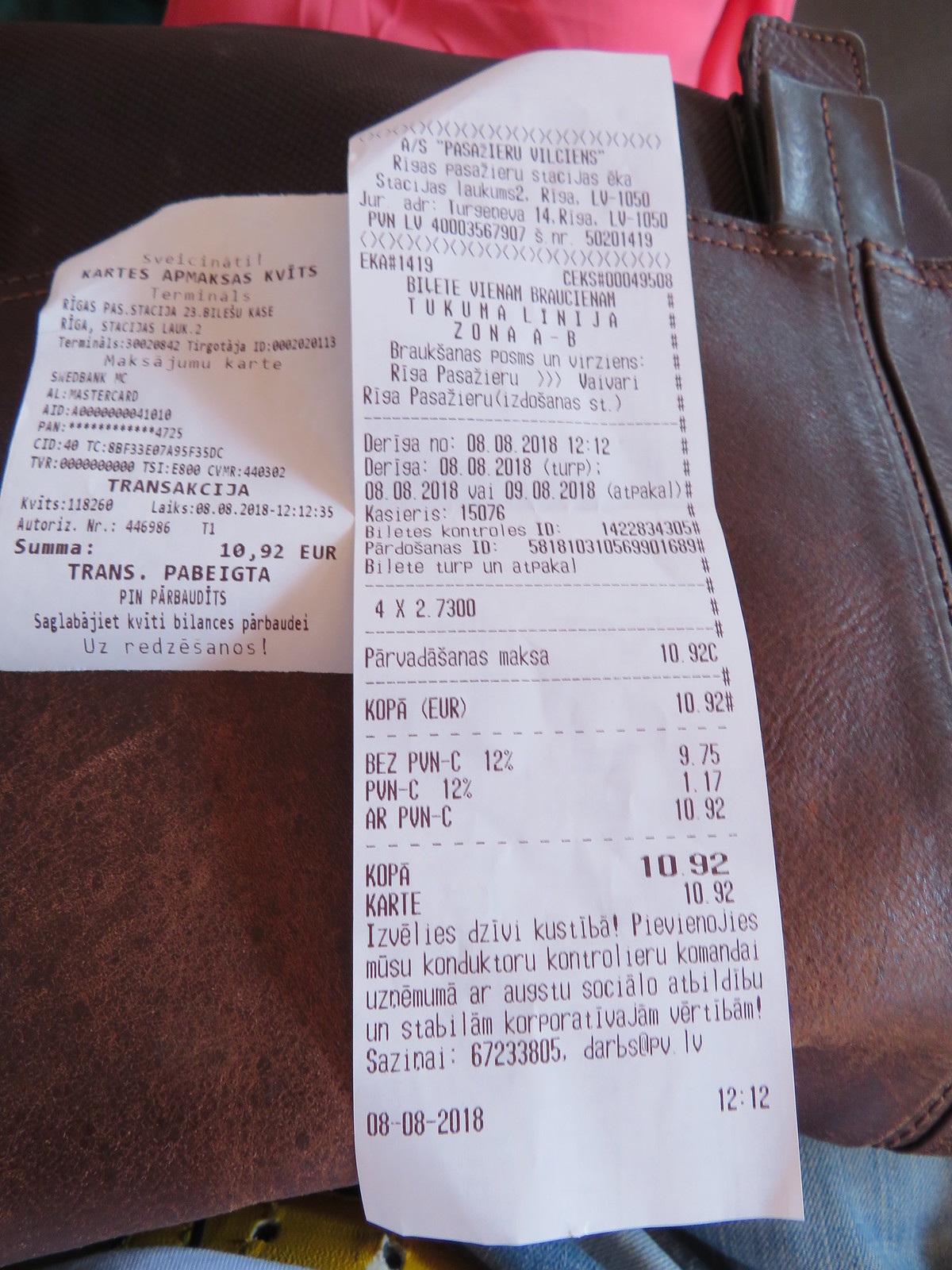The image portrays two distinct receipts side by side. The left-hand receipt is titled "Contest of Boxes Wits," hinting at an intriguing activity or event. Superficially, both receipts resemble typical purchase records one might receive after a transaction. However, a closer inspection reveals that they are printed in an unfamiliar language, suspected to be Greek. This linguistic shift adds an enigmatic layer to the otherwise mundane documents, suggesting that they record participants or transactions related to a possibly intellectual competition.